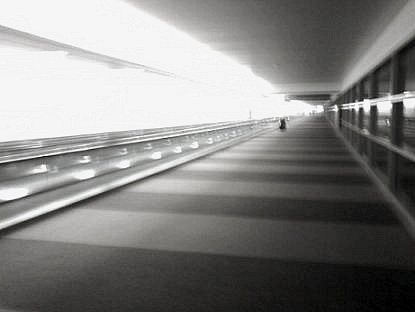This rectangular black-and-white photograph captures a long, enclosed indoor passageway that exudes a sense of ambiguity due to its gray-scale tones and slightly blurred quality. This passageway, potentially part of a subway station or an airport walkway, is framed by a series of distinctive features. On the right-hand side, a row of windows divided into smaller panes, stacking three high, extends down the length of the corridor. The floor is carpeted in a striped pattern, alternating between dark and light bands. The left side of the photograph is characterized by a smooth, white wall topped with a white overhang, possibly housing a series of lights, though these details appear somewhat out of focus. In what could be a conveyor belt or railings suggestive of a transport hub, there's ambiguity about the exact nature of these structures. The far end of the corridor faintly reveals the outline of a solitary figure walking away, enhancing the photograph’s mysterious ambiance. The overlapping elements suggest a clean and orderly environment, despite the blurred nature of the shot, adding to its enigmatic aesthetic.